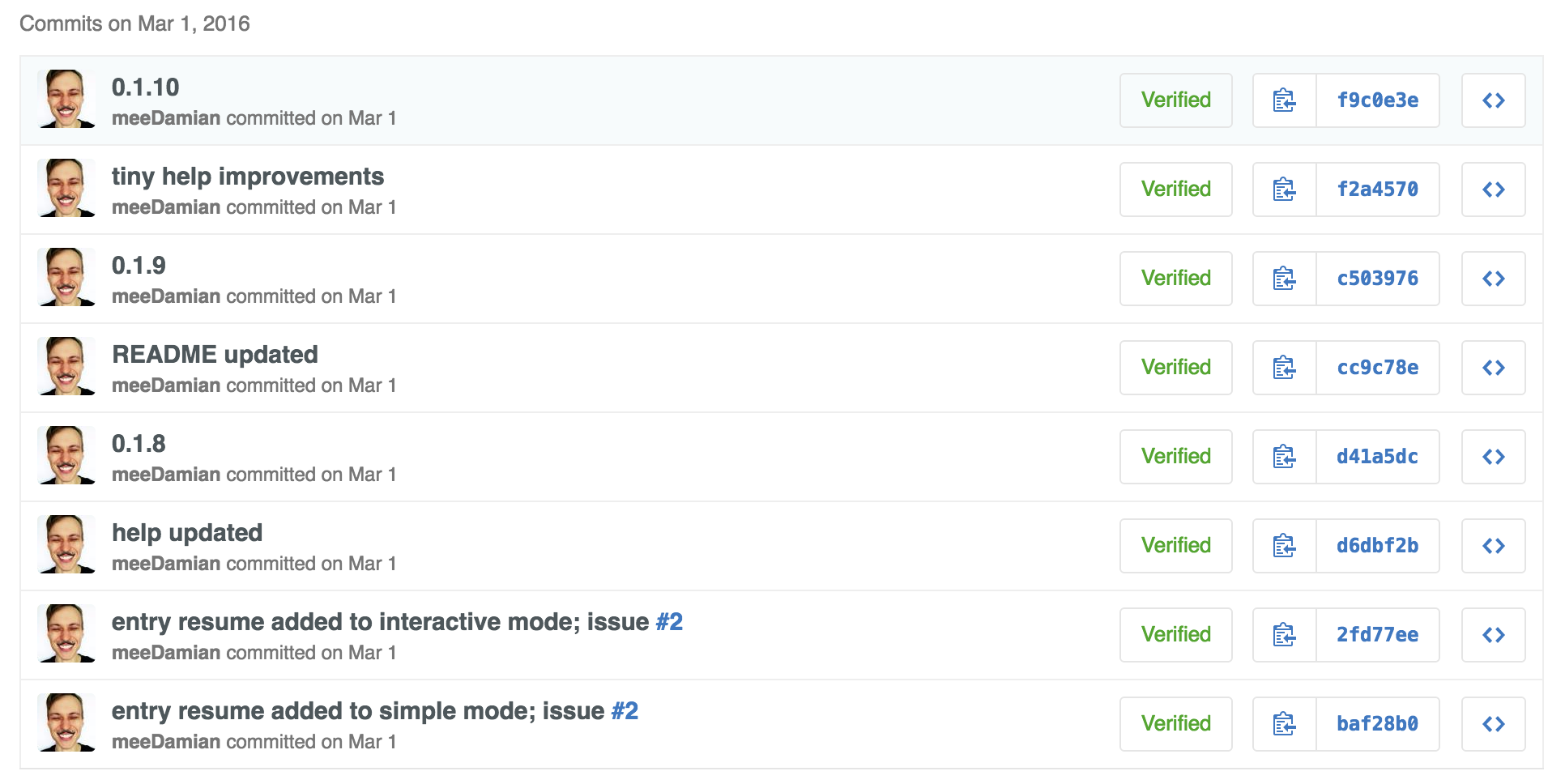Screenshot of a Computer Displaying Commit History

This image is a horizontal screenshot taken from a computer screen, showcasing a commit history. The background is predominantly white. The display contains eight horizontal rows, each delineated by lines spanning the width of the image. 

In the top-left corner, the title "commits on March 1st, 2016" is clearly visible. Each row features a small, square picture of the same man eight times, aligned vertically. The man depicted has dark hair and a dark mustache, and he is smiling broadly.

In the first row, the text reads: "0.1.10, me, Damien, committed on March 1st." Towards the right side of this row, there is a green rectangle labeled "verified." Adjacent to this label, there is a clipboard symbol accompanied by a box with an arrow inside it. Next to this symbol, another rectangle contains the hexadecimal number "F9C00E3E".

To the extreme right of each row, a small white box with an arrow pointing leftward and another pointing rightward is present. All eight rows follow this same layout, presenting similar information with minor variations in text.

Overall, the screenshot provides a detailed view of the commit history, emphasizing the repeated elements for each entry, such as the picture, commit message, verification status, and unique hexadecimal identifiers.